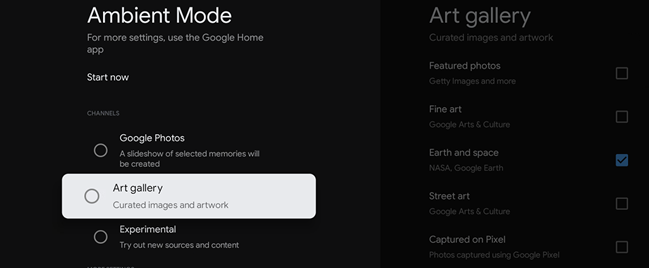The image depicts a screenshot from a device's screen displaying the Ambient Mode settings. The overall background is black, providing a contrasting canvas for the white and gray text. On the left side of the screen, prominently displayed in bold white font, is "Ambient Mode". Directly beneath this, in smaller gray font, it reads, "For more settings use the Google Home app." Below this instruction, there is some space followed by a bold white "Start now" button. Further down, in much smaller gray text, is the label "Channels".

The bottom section of the screen presents three clickable options: "Google Photos", "Art Gallery", and "Experimental". The "Art Gallery" option, which displays "Curated images and artwork" in white, has been selected, turning this section into a white rectangle for emphasis. 

To the left of this area, an opened menu under "Art Gallery" reveals further options. "Art Gallery" is written in gray at the top, with "Curated images and artwork" in a slightly darker gray just below it. The menu offers four categories for selection: "Featured Photos", "Fine Art", "Earth and Space", and "Street Art", along with a fifth option, "Captured on Pixel". Currently, the only selected category is "Earth and Space," indicated by a blue box with a black check mark next to it.